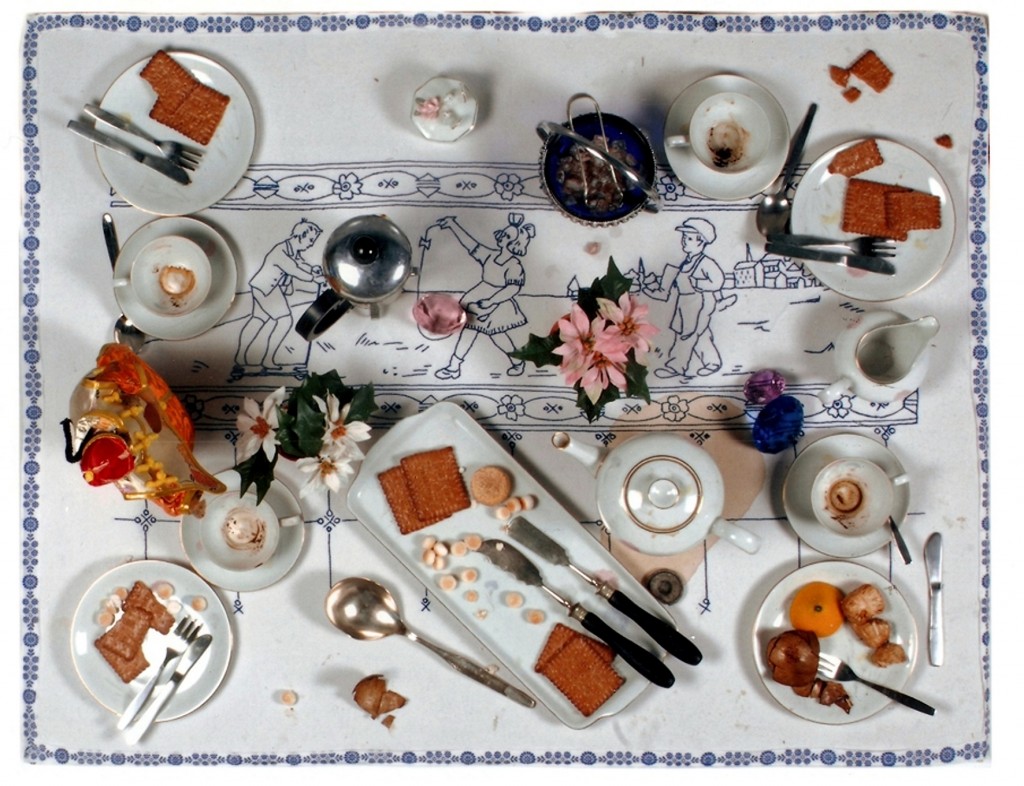This overhead shot captures an elegantly set tea party with a white ceramic platter adorned with various plates of treats, meats, cheeses, chocolates, crackers, and a whole orange. The largest platter is rectangular, surrounded by an array of mostly circular plates, all featuring playful blue accents. Scattered among the plates are utensils including spoons, forks, and knives, as well as little teacups, some showing signs of past use with tea or coffee stains. The scene is further decorated with flowers and set against a backdrop featuring an intricate blue and white pattern with line art of three people playing in the fields. This entire setup is laid on a beautifully patterned tea party blanket or table placemat, framed by elegant curved borders. The colors in the image are predominantly whites, blues, with touches of red, pink, and gold, adding to the festive and refined atmosphere.